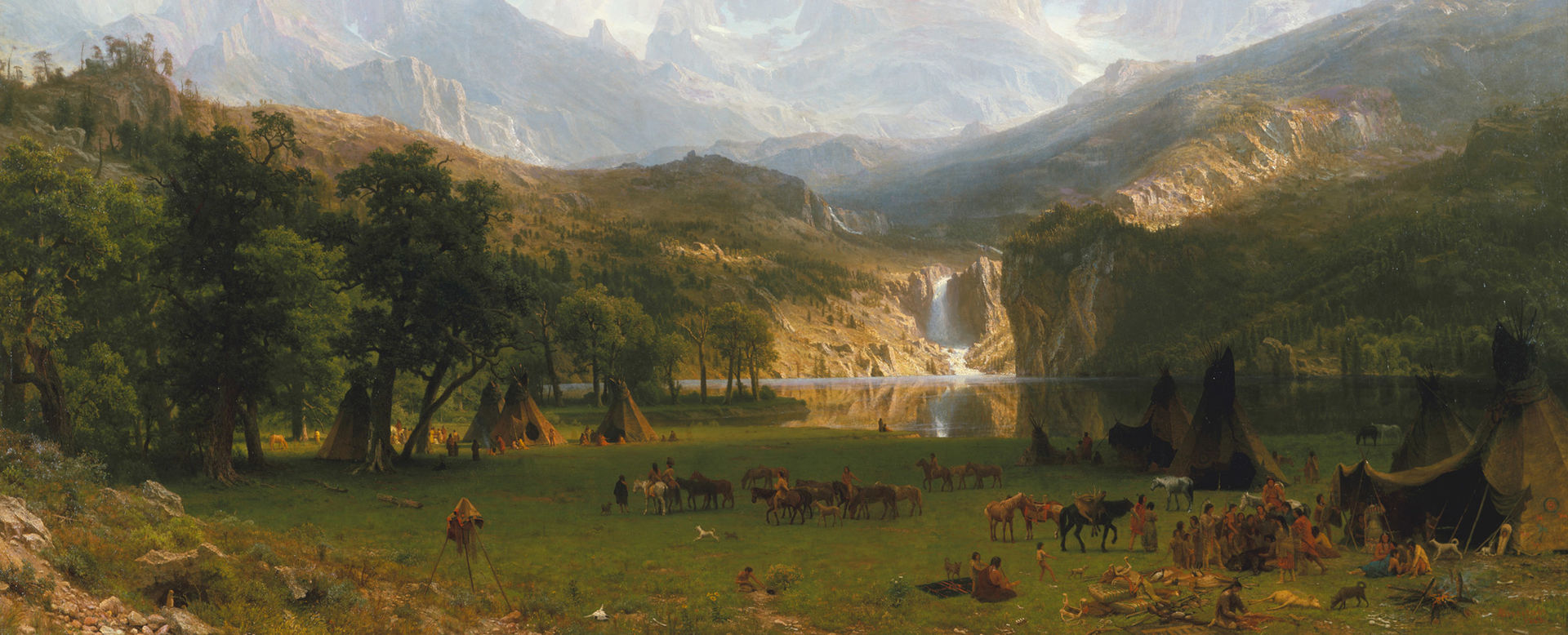The image is a detailed color painting from the 18th or 19th century depicting a serene Native American village set within an unspoiled natural landscape. The scene is vibrant and features several brownish teepees spread out across both the left and right sides near the center of the frame. Numerous Native Americans are seen outside the tents, engaged in various activities. There are also several horses of different colors—brown, white, and black—grazing in the green grassy valley at the front of the painting.

In the background, a tranquil lake with calm, reflective water sits beneath a dramatic rock formation, from which a white waterfall cascades down into the lake. Hillsides, covered with mature dark green trees, slope toward the waterfall on either side, while further in the distance, a range of light gray mountains with a few snow-capped peaks rise majestically.

The painting captures the essence of the daytime outdoor scene with a diverse palette of browns, greens, tans, beiges, blacks, and whites, and it focuses on the harmony between the Native American village and the surrounding wildlife and landscape. The overall composition eloquently portrays a peaceful coexistence with nature during a time when the land was largely untouched.